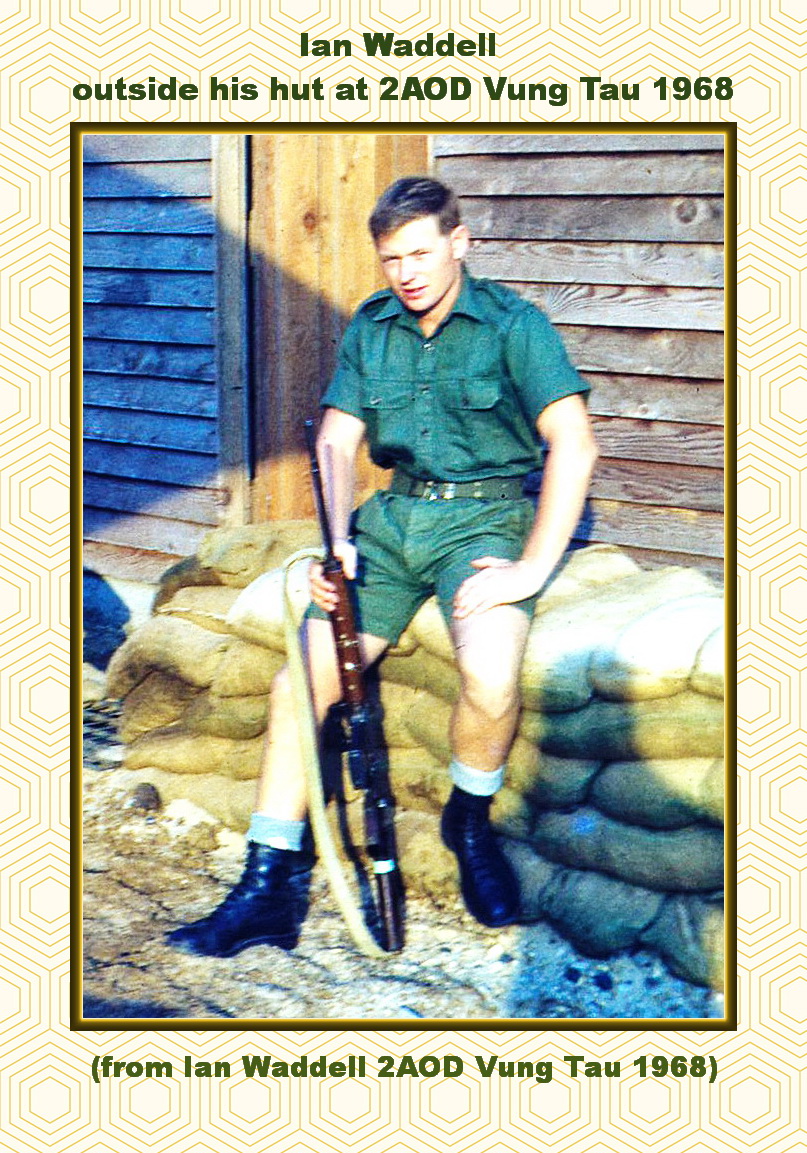The photograph depicts Ian Waddell sitting in front of his wooden hut at 2AOD, Bung Thao (presumably Vung Tau), 1968. He's dressed in a military uniform consisting of a short-sleeved, collared, green shirt tucked into green shorts, and black boots with light green rims. Ian, who is Caucasian with brown hair, holds a rifle with a shoulder strap resting on the ground against his leg while seated on layered sandbags. The photo has a patterned, embroidered background resembling a honeycomb or concentric octagons. The title above the image in green text reads, "Ian Waddell outside his hut at 2AOD Bung Thao 1968," and is repeated at the bottom with the additional note, "From Ian Waddell, 2AOD Bung Thao 1968."